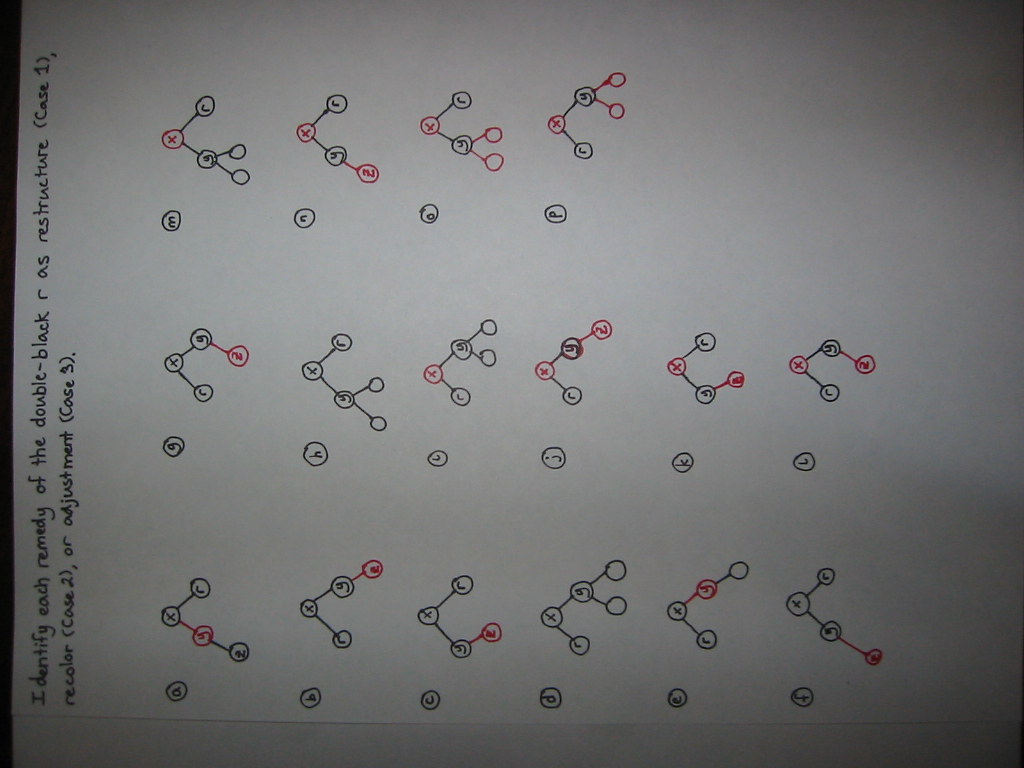The image shows a sideways view of a white piece of paper from an academic study or school project. The paper features intricately drawn molecular structures, illustrating the process of molecular restructuring. Several clusters of molecules are depicted using interconnected red and black circles, with lines denoting bonds between them. Scattered across the page are red and black X's, along with various G's and other alphanumeric annotations within the circles. At the top of the page, there is a prominent note that reads, "Remedy of the double black R as restructure." This indicates a focus on the method of reorganizing molecule structures, or possibly cellular structures. The page is filled with detailed diagrams and annotations, making it a comprehensive guide or study on the molecular or cellular restructuring process.